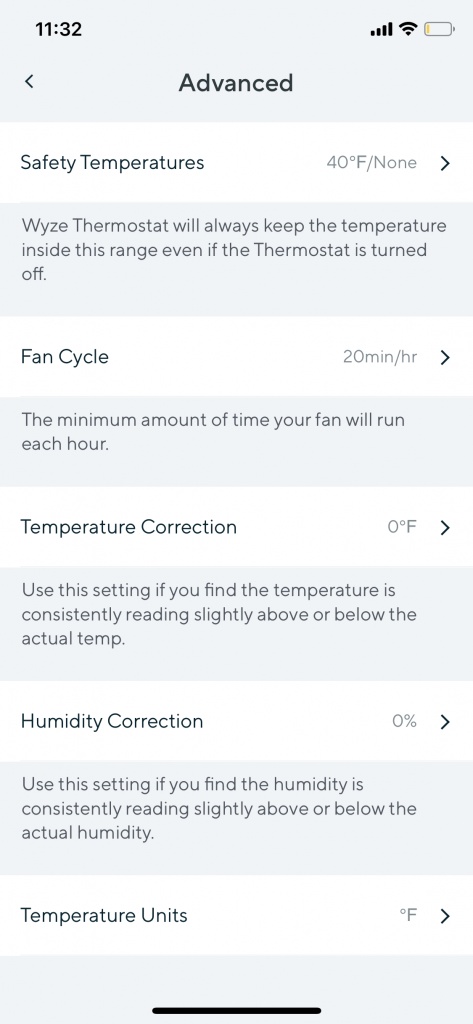**Detailed Caption for Image:**

The screenshot features a white background and showcases a thermostat interface with essential settings and information.

- **Time Advancement**: The current time displayed is 11:32.
- **Safety Temperature Range**: The safety temperature is set at 40 degrees Fahrenheit, ensuring the thermostat maintains the indoor temperature within this range, even when turned off.
- **Visual Elements**: Alternating blue and white rectangles represent different settings.
- **Fan Cycle**: One white rectangle displays "Fan Cycle: 20 HR" (20 hours), marked with a right arrow at the end. This indicates the duration for each fan cycle.
- **Fan Runtime**: A blue rectangle specifies "The minimum amount of time your fan will run each hour."
- **Temperature Correction**: Another white rectangle shows "Temperature Correction: 0 degrees F," with a right arrow, recommending adjustments if the temperature reading consistently deviates from the actual temperature.
- **Humidity Correction**: Similarly, a white rectangle reads "Humidity Correction: 0 percent," providing guidance to align humidity readings with actual levels.
- **Temperature Units**: Finally, another white section indicates the temperature units as "0 degrees F."

This detailed image is designed to help users fine-tune their thermostat settings for optimal performance and accuracy.